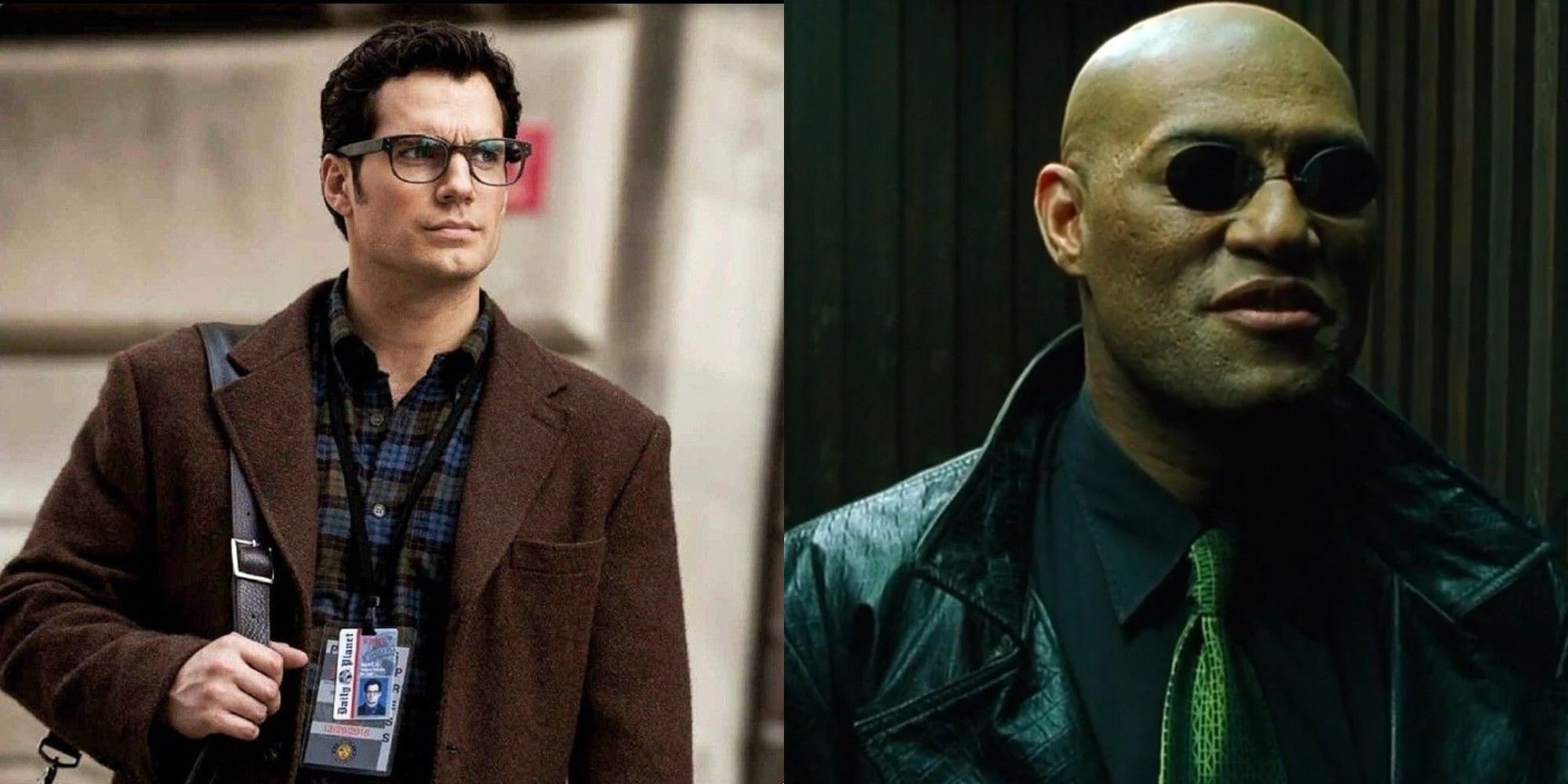The image features two distinct movie actors portrayed in color photos side by side. On the left, Henry Cavill, believed from his role as Superman, stands against a backdrop of what appears to be a concrete building. He exhibits a serious expression with large black glasses and dark, slightly fluffed hair with sideburns. He has a pronounced cleft chin and a slight tan. Cavill is dressed in a brown jacket with a plaid shirt underneath, likely brown, blue, and black. Around his neck, he sports a lanyard with press credentials, presumably identifying him as Clark Kent, and slung over his right shoulder is a leather satchel.

On the right, Lawrence Fishburne is depicted in character from the Matrix series, recognized for his role in teaching Neo. He has a bald head and wears distinctive dark glasses that lack temples, sitting directly on his nose. Fishburne's attire includes a black leather jacket over a blue shirt and a green tie, aligning with his iconic look from the Matrix franchise.